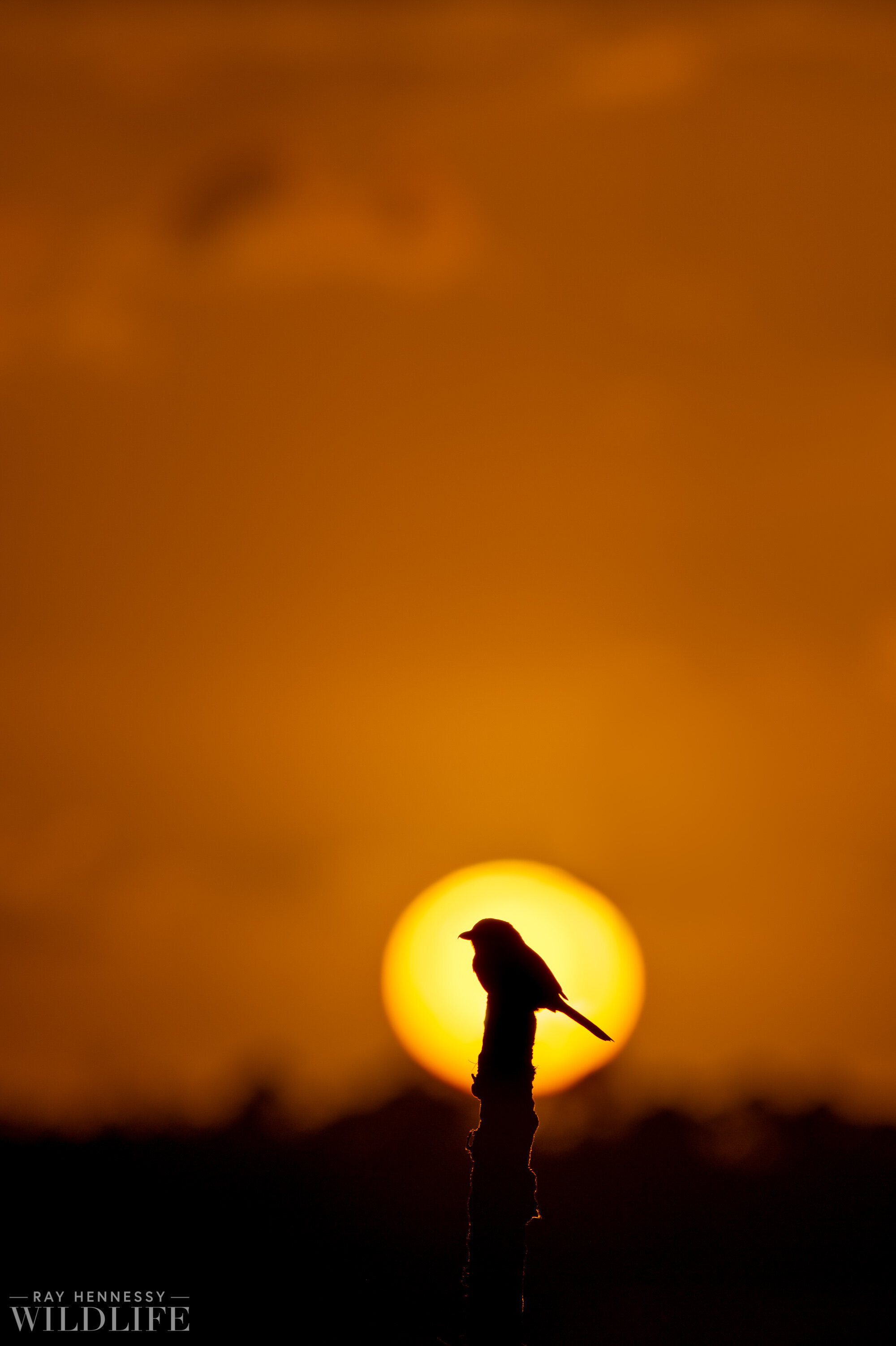This evocative photograph taken by Ray Hennessy Wildlife features the striking silhouette of a small bird perched atop a truncated tree or plant. The bird is centrally positioned in the frame, directly aligned with the intensely bright yellow-orange sun, either rising or setting. The sun bathes the scene in a radiant glow, highlighting the bird's detailed silhouette, complete with visible beak and tail. The foreground is shrouded in darkness, likely depicting an indistinct forest or landscape, lending the scene a sense of mystery. From the lower portion stretching to mid-frame is a blur of dark forms, possibly suggesting hills, trees, or structures. The sky above transitions into soft orange hues with faint, blurred clouds, creating an overall muted backdrop. In the lower left corner, "Ray Hennessy Wildlife" is clearly inscribed in a greyish hue, standing out against the dark background, emphasizing the simplicity and focused beauty of the image.